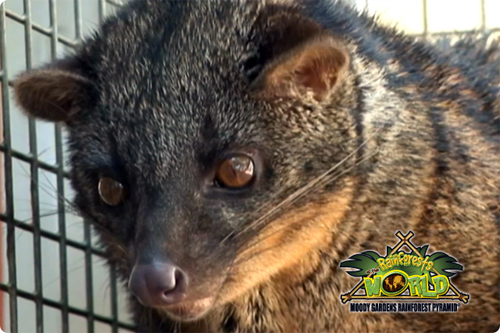The image is a close-up shot of a wild animal enclosed in a cage, focusing on its head and neck features. The animal exhibits a mix of characteristics reminiscent of a possum, raccoon, or perhaps even a small bear, though its exact species is unclear. It has dark brown, cat-shaped eyes and small ears, along with a black nose and long whiskers protruding from its somewhat pointy snout. The fur is a blend of black and brown with patches of tan, appearing thinner around the lower part of its face where the skin turns a brownish hue. The animal's gaze is directed downward, giving it an uneasy appearance, further accentuated by the photograph's close-up nature. Situated in the bottom right corner of the image is a logo reading "Rainforest World, Moody Gardens, Rainforest Pyramid," featuring a pyramid and green leaves.